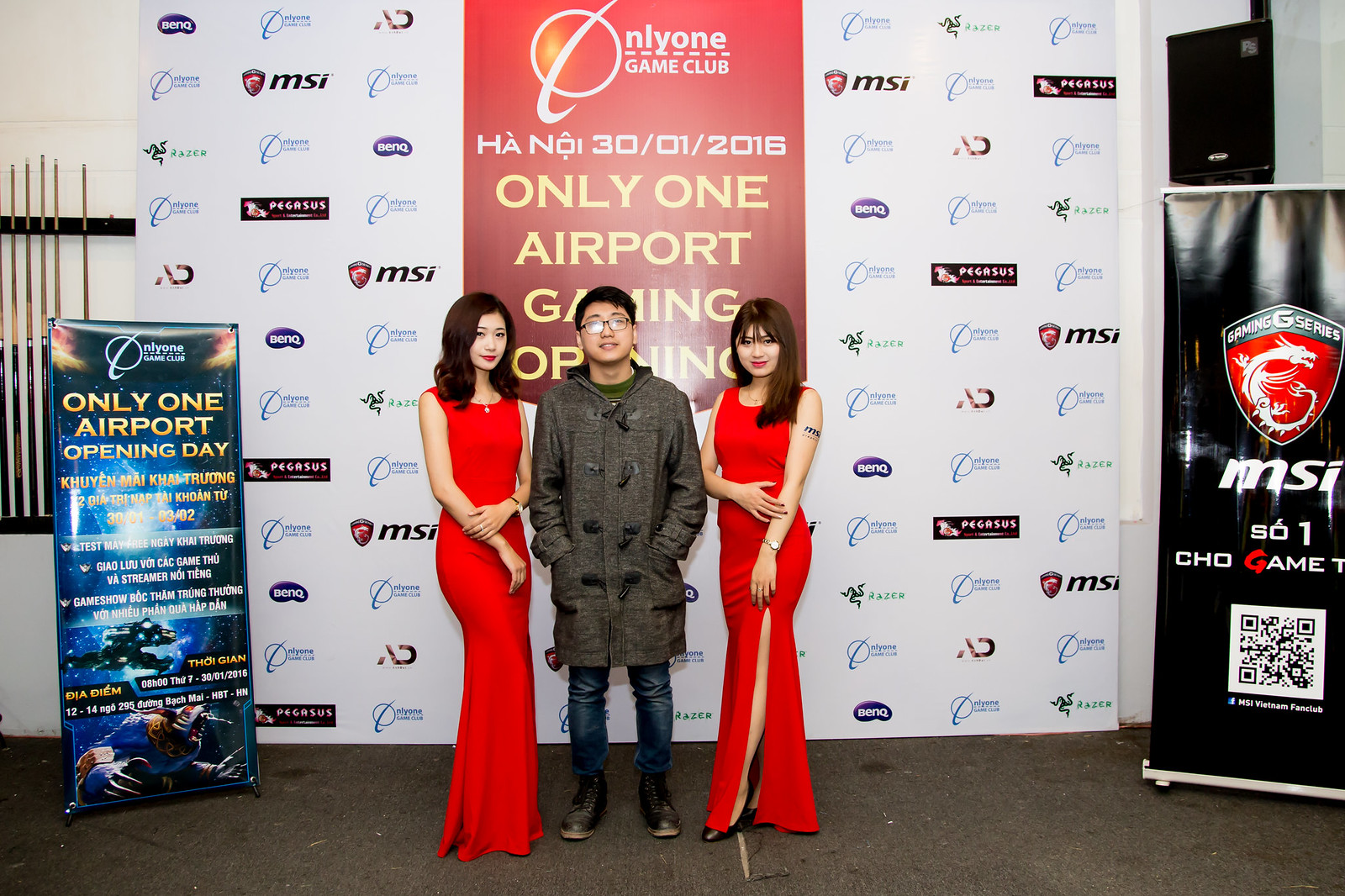In this image, three Asian individuals are pictured at an event which appears to be the opening of a game club, suggested by the banners and signage in the background. These banners include text in a foreign language and phrases such as "Nalai 1 Game Club," "Only One Airport Gaming Opening," and "Only One Airport Opening Day." Prominently featured logos include MSI, Pegasus, and a dragon shield emblem with "Gaming G-Series, MSI, SO1, Show Game." A large banner behind the group displays various logos likely associated with the event's sponsors.

The two women flank the man in the center. Both women are dressed in long, sleeveless red dresses, one of which has a slit up to the thigh. They both have long, brown hair. One woman, positioned to our right, sports a watch and has a visible tattoo on her arm. The man between them is casually dressed in blue jeans, black boots, a green shirt, and a long grey trench coat with a hood. He has short black hair, glasses, and is smiling for the photo.

The overall setup suggests a vibrant atmosphere, possibly in an Asian country, given the participants and language on display. The background includes a yellow and white poster with text too distant to fully decipher and a floor poster further emphasizing the "Only One Airport Opening Day" theme, enhancing the gaming event's official and festive ambiance.